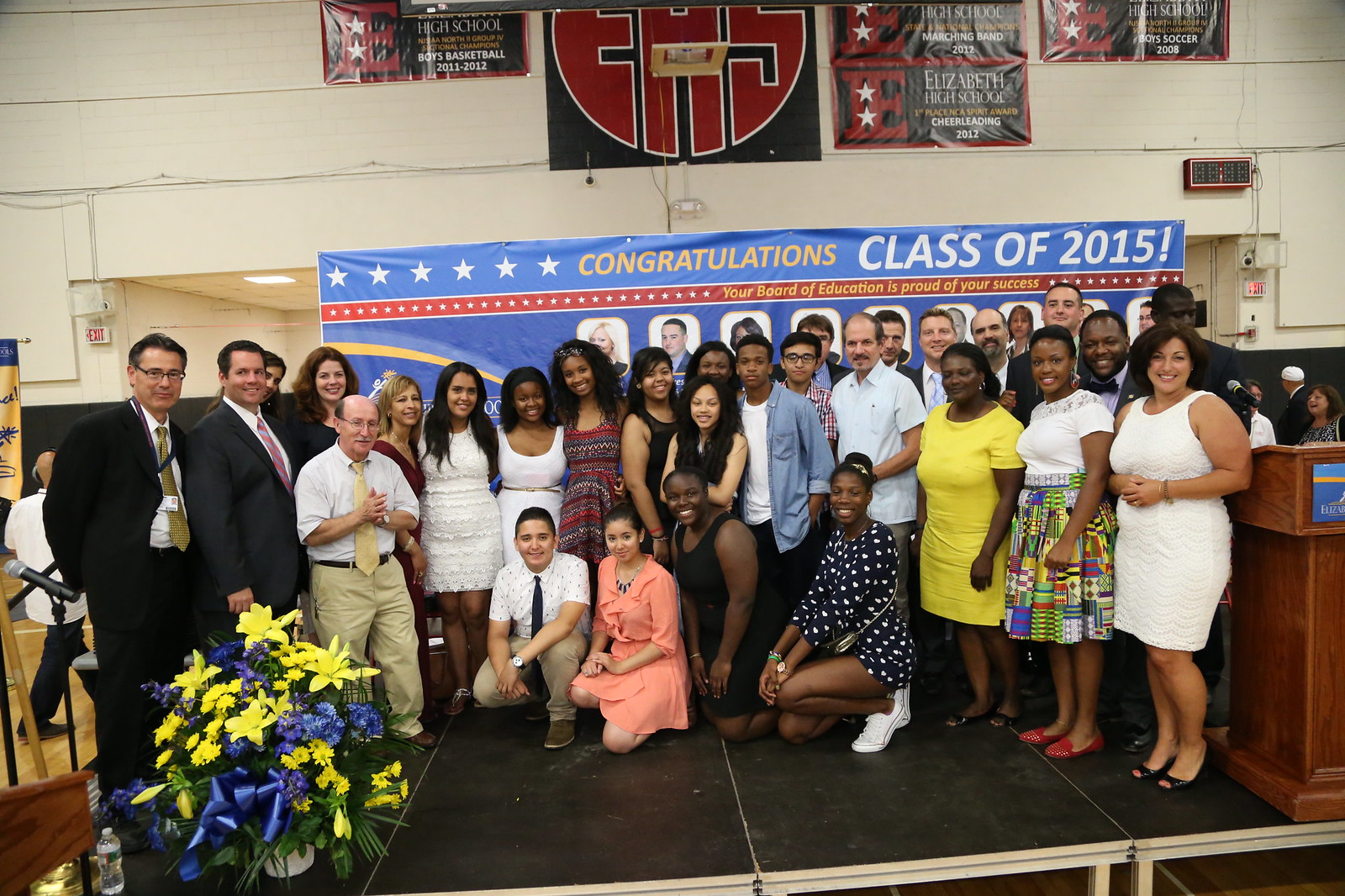The image captures a group of approximately 30 young people, primarily women, who appear to be graduating high school students, posing for a group photo in what seems to be a gymnasium. Behind them is a prominent blue banner with gold lettering that reads, "Congratulations, Class of 2015. Your Board of Education is proud of your success." This central message suggests a high school graduation. 

The background features white panels and several banners, including those for boys' basketball (2011-2012), marching band (2012), cheerleading, and state national champions for boys' soccer (2008). These banners, although somewhat difficult to read, celebrate the school's various achievements. 

The group is gathered on a platform, with a podium visible on the far right of the image. The students are surrounded by a few adults who are likely faculty or school officials, including one in a suit and another in a short-sleeved shirt and yellow tie. 

A bouquet of yellow and blue flowers and a bottle of water adorn the lower left corner of the photo, adding a touch of celebratory decor. The students and faculty members are all smiling, exuding a sense of accomplishment and joy, epitomizing the spirit of graduation.